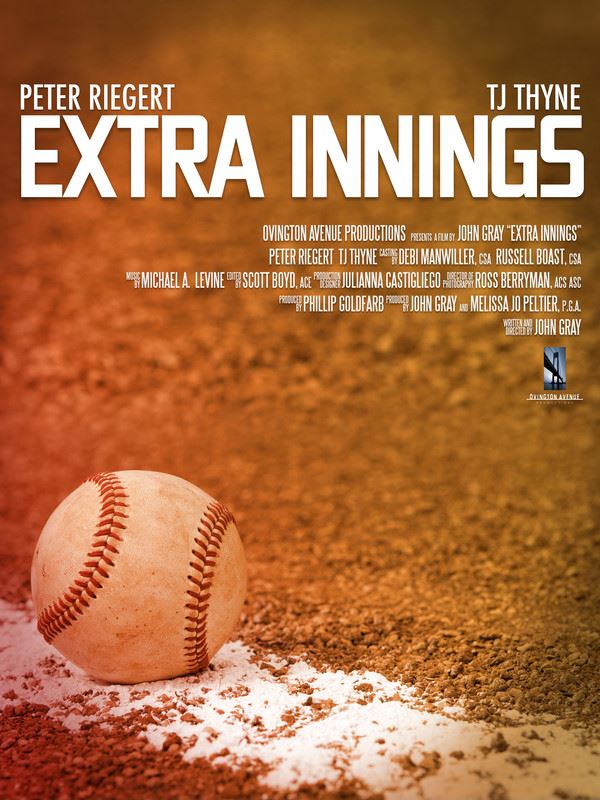This movie poster for the film "Extra Innings" prominently features a dirtied baseball resting on the white foul line of a baseball field. The image has a reddish-brown hue, giving it a warm, nostalgic feel. At the top left of the poster, the name Peter Riegert is displayed in white font, mirrored by T.J. Thyne's name on the top right. The film's title, "Extra Innings," is boldly written in large white letters across the center of the poster. Below the title, the poster credits Ovington Avenue Productions and mentions the film's director, John Gray. Further down, it lists the casting done by Debbie Manwiller, CSA, and Russell Boast, CSA, along with a variety of other producers and contributors in smaller white text. The design effectively captures the essence of a classic baseball game and sets the scene for the film's themes.